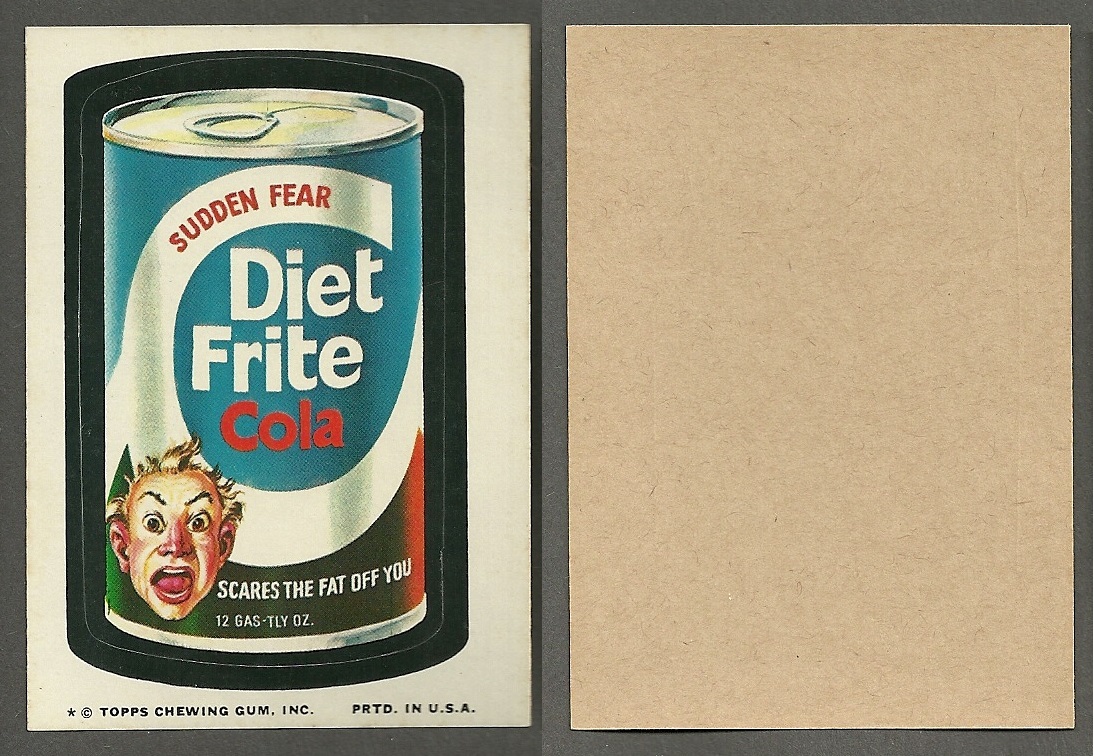This image features a vintage-style advertisement card with a humorous yet eerie theme. The ad is designed as a bifold card with a gray border, folded down the center, resembling a greeting card. On the left panel, there is an artistic depiction of a can labeled "Diet Fright Cola," predominantly colored in light blue and white. The word "cola" is written in striking red letters. The top section of the can proclaims "Sudden Fear" and "Diet Fright" (spelled F-R-I-T-E) in white print. Below this, it reads "Scares the Fat Off You" and states "12 ghastly ounces." An unsettling, shocked-looking man with unruly hair is illustrated on the can's lower left side. The card credits "Topps Chewing Gum, Inc." and notes that it was "Printed in the USA." The right panel of the card is a plain, tan sheet, indicating that the card can be closed after viewing the advertisement.